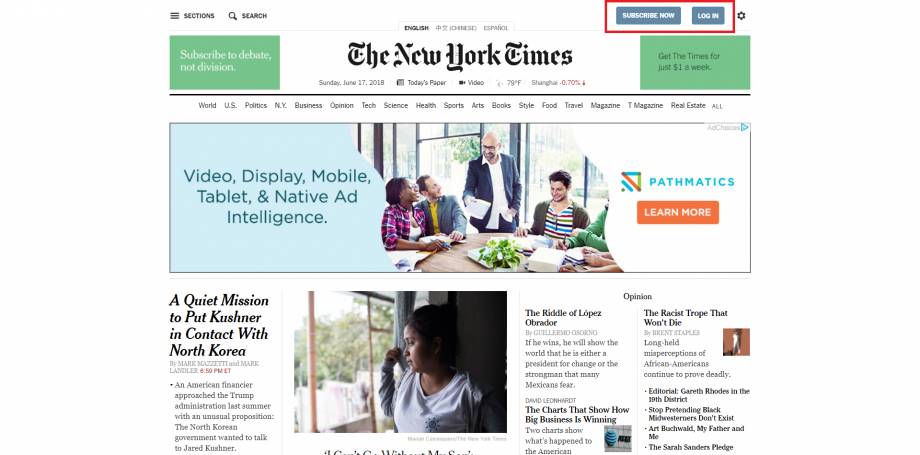The screenshot features the New York Times website, showcasing its iconic name and logo at the very top, rendered in elegant black calligraphy using the Times Roman font. On either side of the header are light green boxes; the one on the left displays a message in white text saying "Subscribe to debate, not division," while the box on the right promotes a special offer stating "Get Times for just a dollar a week." In the upper right corner, a red outline highlights two buttons: one for subscribing and another for logging in.

Beneath the header is a prominent display advertisement. The ad has a blue background on the left side, with the text "Video Display Mobile Tablet Native Ad Intelligence." Central to the ad is an image of a roundtable discussion featuring four individuals: a Black woman seated on the left next to a White man. Another White man, bald with a mustache and beard, dressed in a white shirt and blue jacket, sits next to a third White man, who is wearing a striped shirt. Additionally, a figure with green sleeves is partially visible to the right.

At the very bottom, there is a news article headline on the left side that reads, "A quiet mission to push Kushner in contact with North Korea," accompanied by a photo related to the article.